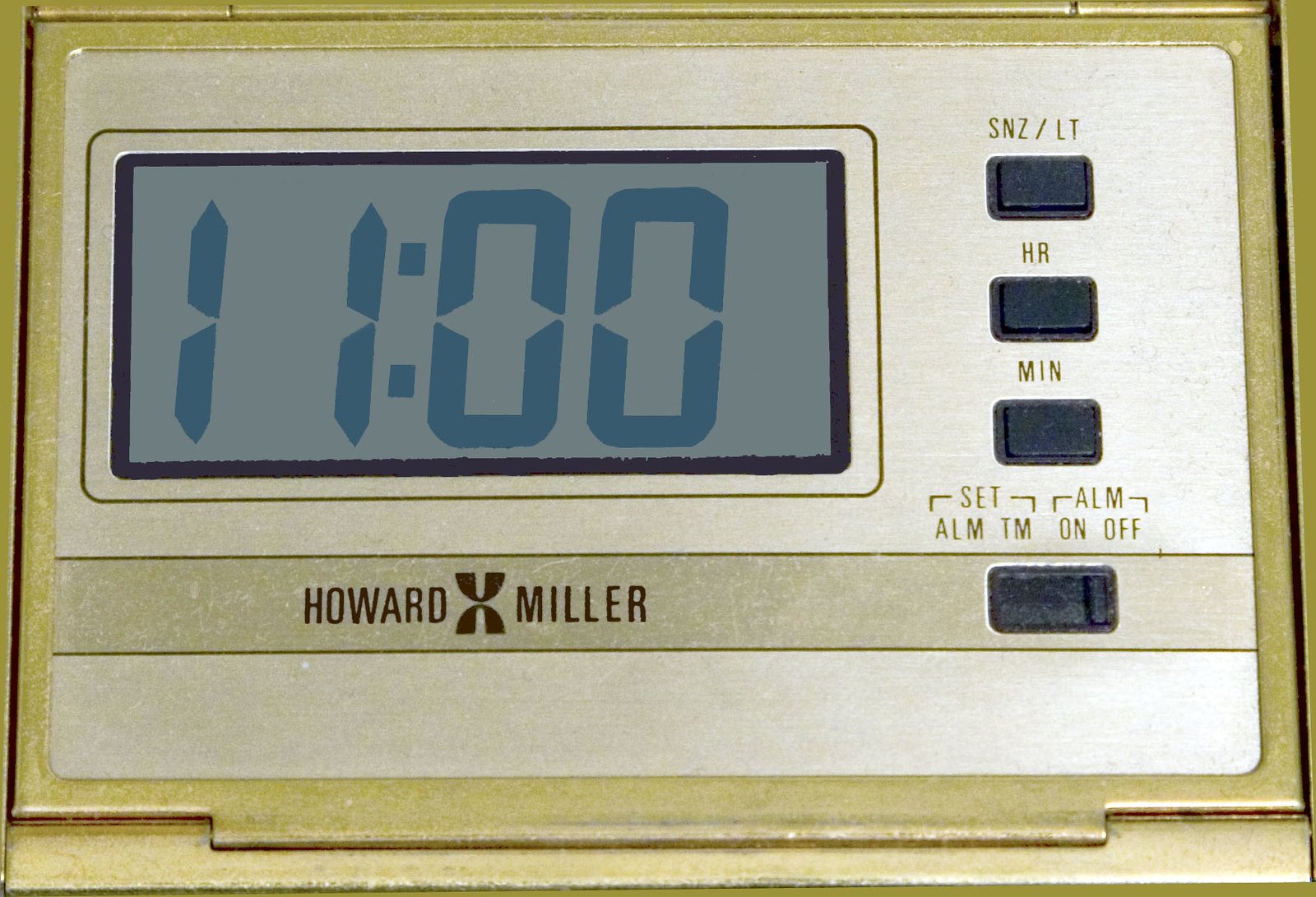The image showcases a retro-looking alarm clock with a digital display reading "11:00." The clock features a rectangular design with gold, faded gold, and bronze trimmings that frame its face. The digital display, which is set within a silver border, prominently shows the time. Centered on the silver border is the brand name "Howard Miller," with 'Howard' on the left and 'Miller' on the right, intersected by a decorative element resembling an "X." 

Right of the display, several black buttons can be seen. The top button is marked "Snooze/LT," the middle buttons are labeled "HR" (hour) and "MIN" (minute), and the bottom button is for setting alarms. Additionally, there is a switch to toggle between setting the time (TM) and the alarm (ALM), with positions to turn the alarm on or off. The clock's design is further highlighted by a hinge at the bottom, accentuating its vintage aesthetic.